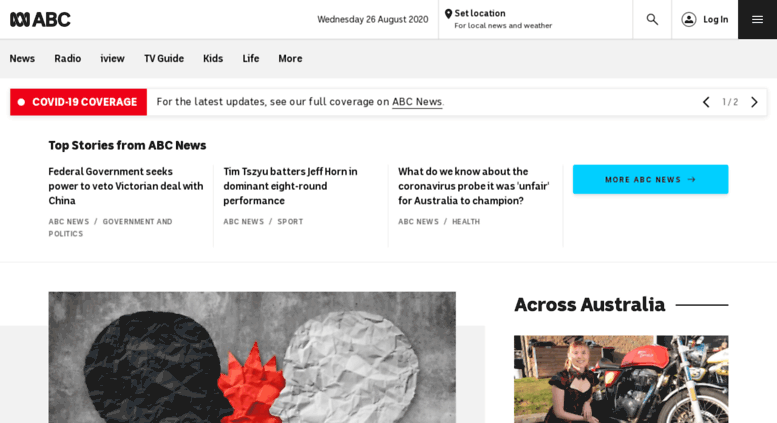Title: ABC News Screenshot Overview - August 28, 2020

In the upper left corner of the image, the iconic ABC logo is prominently displayed. Just below the logo, the image indicates the date, "Wednesday, 28 August 2020," signaling the day's information. A search icon, a login option, and a menu icon represented by three white lines stacked on top of each other are situated towards the right.

The primary section of the image is dedicated to various navigation options: "News," "Radio," "iView," "TV Guide," "Kids," "Life," and "More." Beneath these categories, there's a special notification: "COVID-19 Coverage - For the latest updates, click here." Directly underneath this message, there are navigation arrows on the right side allowing users to move left and right between different sections.

One of the highlighted areas features "Top Stories from ABC News," with a headline stating, "Federal Government Seeks Power to Veto Victorian Deal with China." Another primary story mentions "Tim Tszyu batters Jeff Horn in a dominant eight-round performance." In addition, there is an inquiry about the fairness of the coronavirus investigation towards Australia.

A prominent blue button that says "More ABC News" is provided below these headlines. Further down, there is a section that announces "Across Australia," suggesting more localized news content available for viewing.